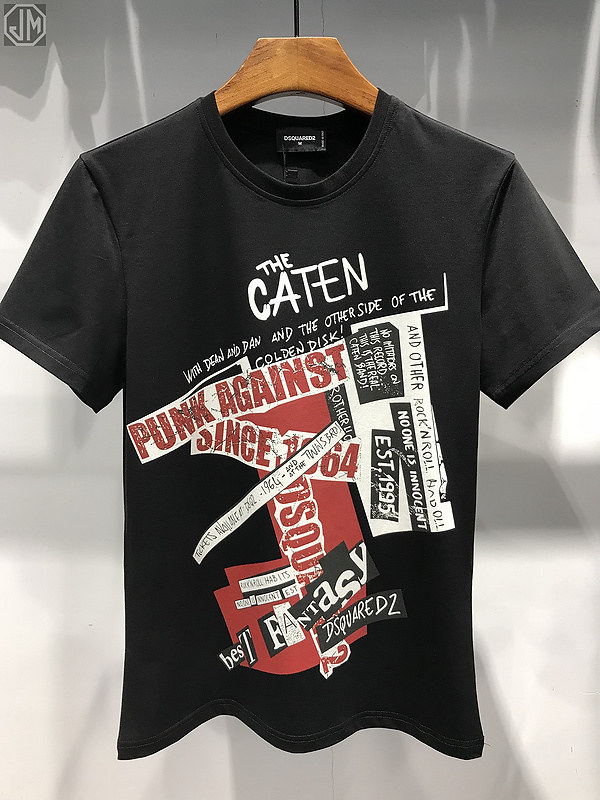The image showcases a black graphic t-shirt hanging on a light brown wooden grain hanger with a black hook. The background is a stark white, casting shadows of the shirt and hanger onto the wall behind it. At the top of the image, there's an octagonal logo with a white exterior and a black interior, displaying the text "JM" in white within the black section.

The t-shirt features a variety of bold, cutout-style texts and slogans across its front, giving it an edgy, punk rock aesthetic reminiscent of Persona 5's graphical style. Prominent among the lettering, the top line in white text reads "the CATEN," spelled "C-A-T-E-N," positioned at a slight diagonal. Below that, in a similar slanted fashion, are fragments of other texts, including references like "the other side of the golden disk," "Dean and Dan," and "the Canteen." 

One standout rectangular white patch bears the red text "PUNK AGAINST," angled opposite to the word "SINCE," followed by the partially legible "1-something-6-4," hinting at the year 1964. Additional phrases and slogans such as "Best Fantasy," "D2," and "No one is innocent" contribute to the shirt's rebellious theme. The scattered typography in white, black, and red contrasts sharply against the black fabric, making each word and phrase a striking element of the design. Established in 1995, this dynamically designed tee embodies a fusion of rock and roll and punk influences, celebrating a gritty, underground culture.